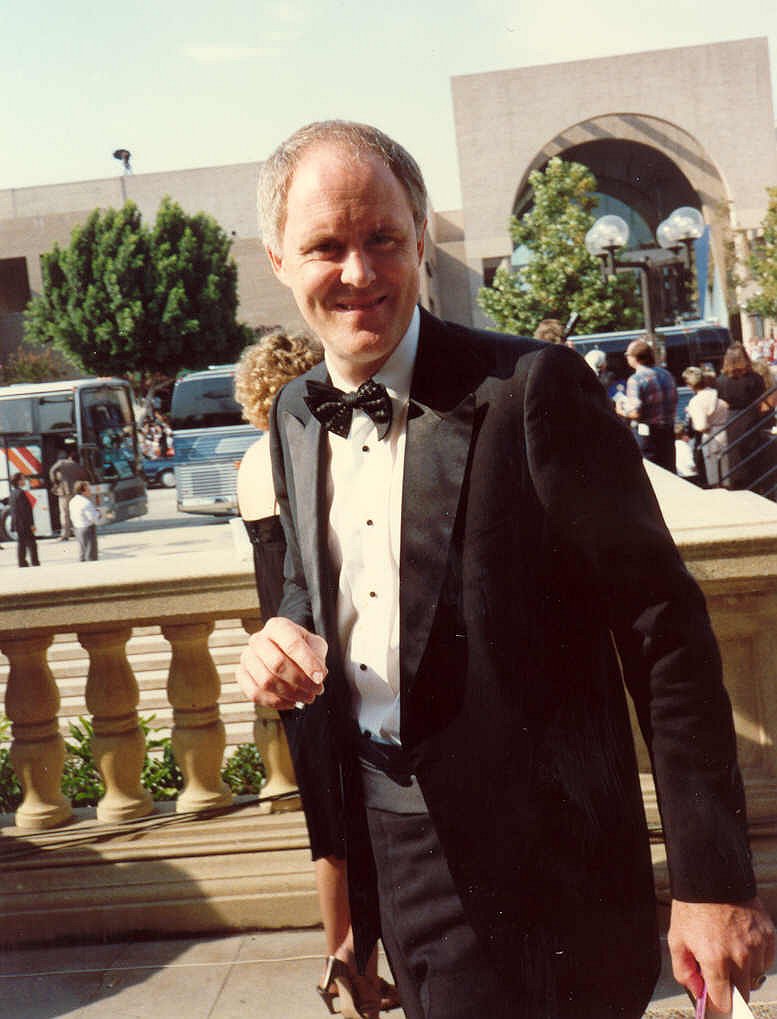The image captures a lively outdoor scene featuring a man dressed in a sharp black tuxedo with a white dress shirt, black buttons and collar, and a distinctive black bow tie adorned with gold polka dots. He completes his formal attire with black dress pants, a black cummerbund, and a black leather belt. Smiling and looking ahead, he walks along a tiled walkway, his left hand holding an indistinguishable item. The setting exudes a vintage vibe, enhanced by a yellow filter that makes the photograph feel aged. This outdoor setting is bustling with activity, as visible behind the man is a woman dressed in a thigh-length black dress and silver high heels, looking in the opposite direction. Further back stands a low ledge with Roman-style pillars, barely reaching hip height, beyond which a busy road lined with trees and a streetlamp stretches out. The road hosts various vehicles, including buses, and teems with people, capturing the essence of a vibrant day under a clear blue sky.